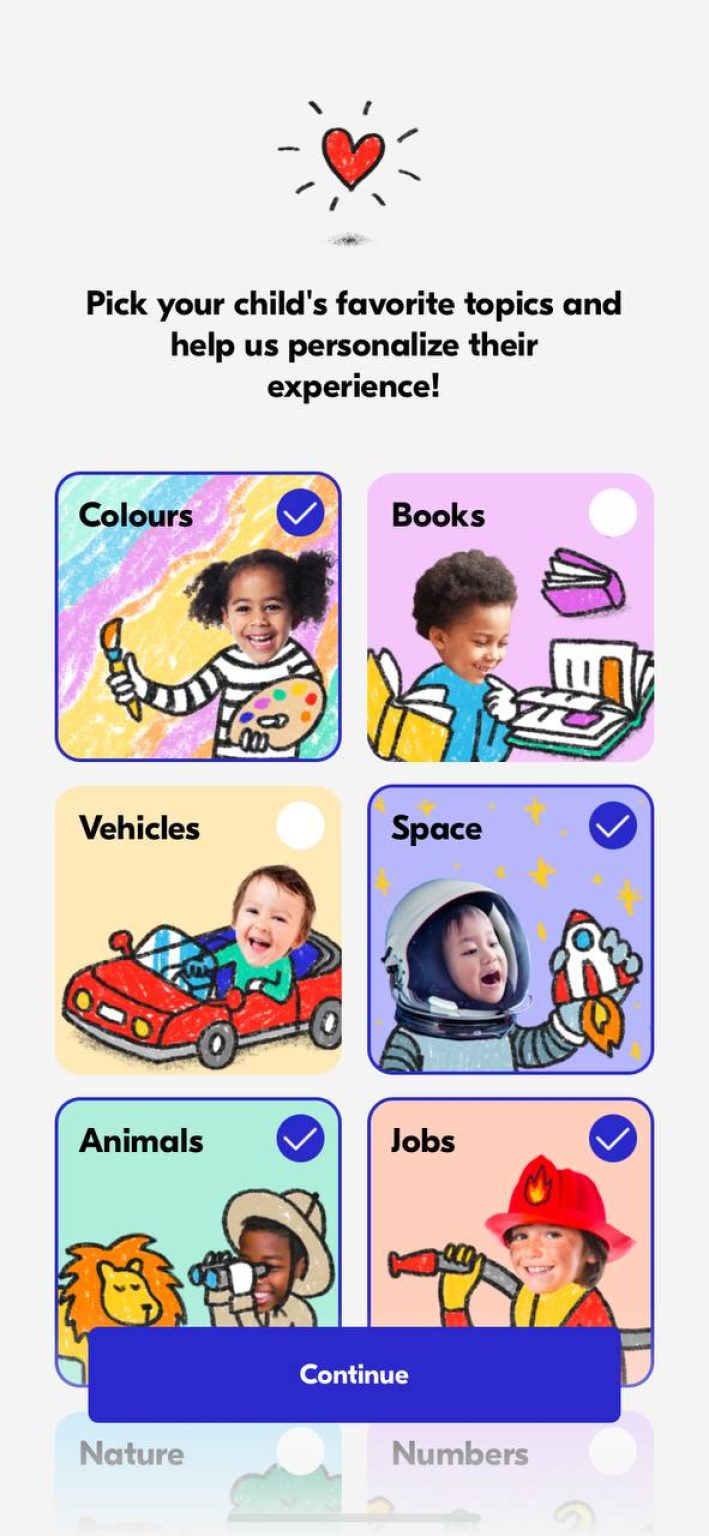This appears to be a vibrant and engaging educational website aimed at very young children, particularly toddlers and kindergartners. The webpage features a gray background with a hand-drawn red heart outlined in black situated at the top center, accompanied by decorative lines around it. Beneath this, a message in black text reads, "Pick your child's favorite topics and help us personalize their experience."

Further down the page, there are six colorful squares representing different topics, designed to attract young users with their playful aesthetics. Each square has a distinct colored background and is labeled with black text in the top left corner indicating the topic. Additionally, each square features an illustration of a child with a cartoon body performing an activity related to the topic, surrounded by themed objects:

1. The first square, labeled "Colors," showcases a girl with a cartoon body painting against a rainbow background.
2. The second square, labeled "Books," depicts a child with a cartoon body engrossed in an open book, surrounded by numerous other books on a purple background.

The layout hints at more squares below, partially visible, suggesting additional topics to explore. Overall, the website aims to create a personalized educational experience for young children by letting them choose their favorite topics through visually appealing and interactive elements.